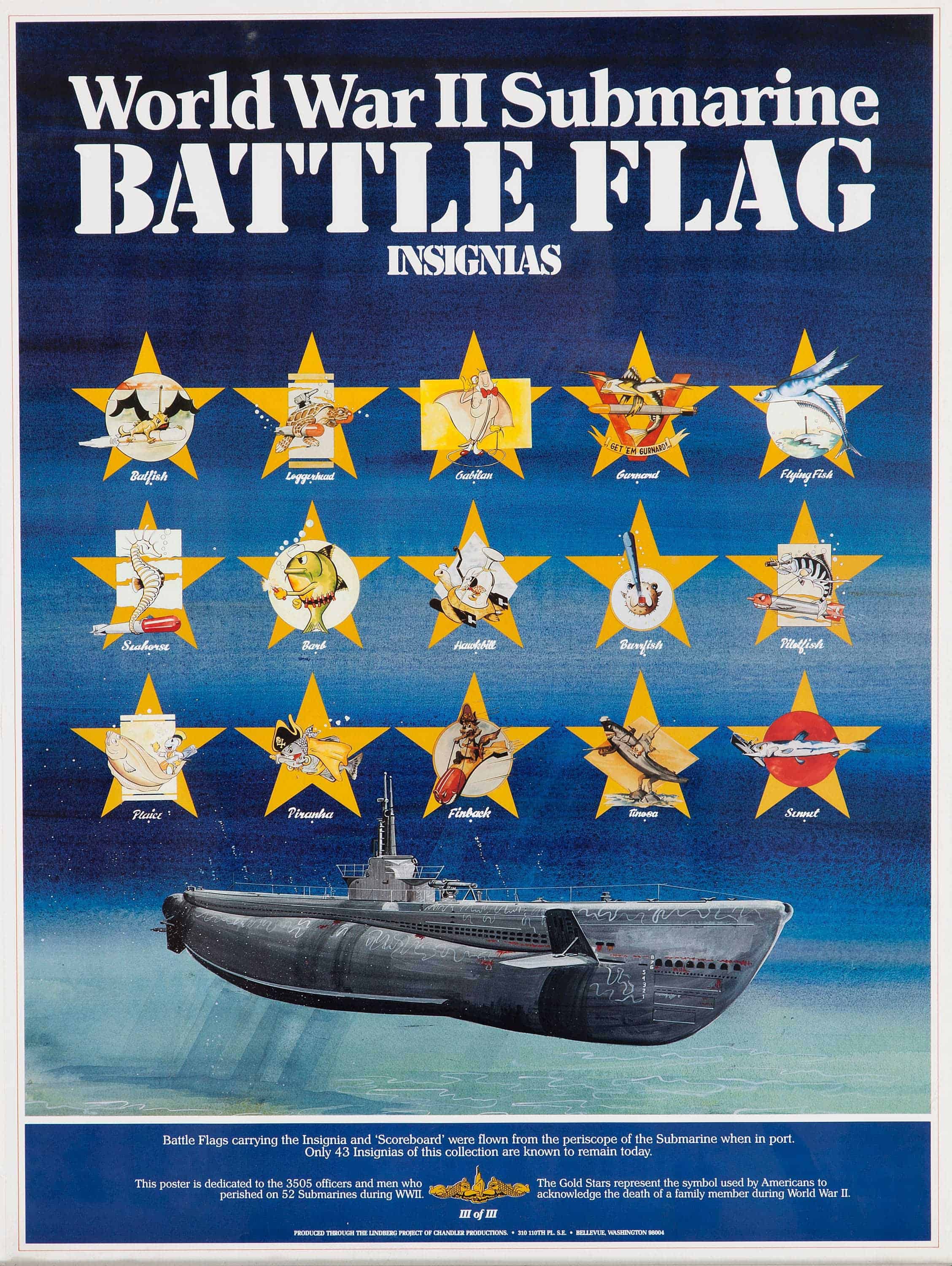The poster, framed in white and set against a multilayered blue ocean background, prominently displays the title "World War II Submarine Battle Flag Insignias" in large, white block letters at the top. Beneath this text are 15 yellow stars, each featuring a unique battle flag insignia, some showcasing red or blue colors, fish, a seahorse, and various other designs. Each insignia is printed over its respective gold star, creating a striking visual effect. Below these stars, an illustrated dark gray submarine with a prominent conning tower is depicted, appearing to face the viewer as if underway. The bottom section features a blue banner, crossed by a thin white line, which contains small, unreadable text along with a central golden naval insignia. The background, designed to represent the ocean with light streaks piercing the water, adds depth and context to the historical theme of the poster.